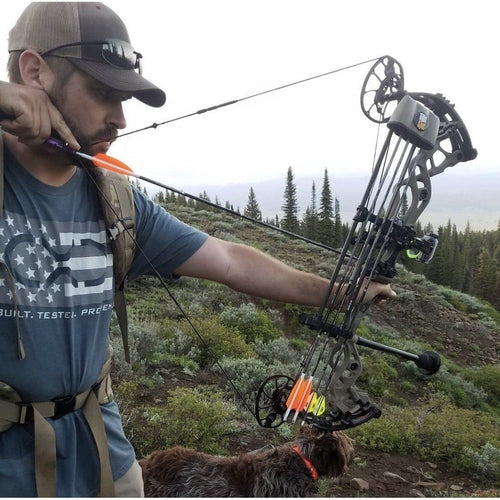This is a detailed color photograph of a man in his 20s or 30s using a mechanical metal crossbow. He is positioned on the left side of the image, looking to the right, with his arm drawn up by his ear, ready to release an orange-tipped arrow. The crossbow has additional arrows stored at the front. The man is wearing a blue t-shirt depicting what seems to be part of an American flag with some unreadable text, and short sleeves. He also has on a gray and white ball cap with sunglasses perched on the brim, a beard, and a mustache. A backpack strap is visible over his shoulder, and he is wearing a belt around his waist. At the bottom of the photo, a brown dog with a shaggy coat and an orange collar stands beside him on some tiny rocks. The background features a green rolling hill, trees, and possibly mountains cloaked in fog or clouds, indicating a cloudy day.